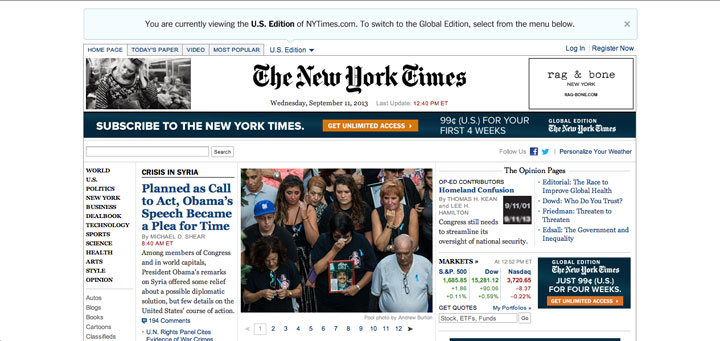This screenshot captures the homepage of the New York Times dated September 11, 2013. At the top, the classic New York Times logo is prominently displayed alongside a navigation bar featuring options such as Homepage, Today's Paper, and Video. This is the U.S. edition, with a prompt for readers to switch to the Global Edition. 

The main headline addresses the Syrian crisis, highlighting President Obama's speech with the title "Planned as Call to Act, Obama's Speech Became a Plea for Time." Below this headline, there is a poignant photograph of a woman crying in public, credited to Andrew Burton of Getty Images. 

In the lower left-hand corner, stock market values for major indices like the S&P 500, the Dow, and the NASDAQ are noted. Below the main content, additional navigation options are visible, including categories such as politics, world news, and other current events, offering readers easy access to a variety of news topics.